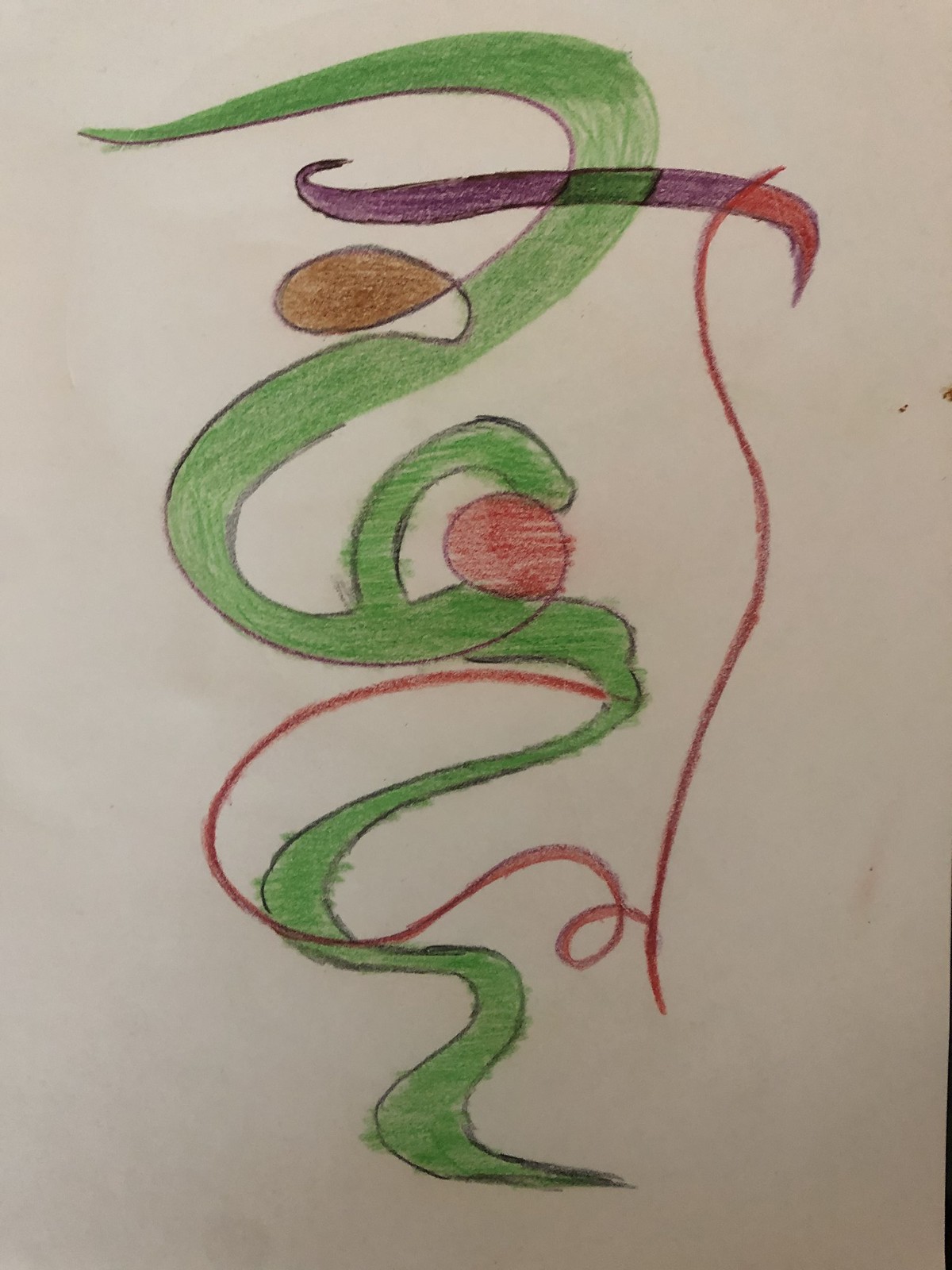This crayon drawing is rendered on white sketch paper and prominently features two large, green "2" shapes aligned vertically, one above the other. At the top of the image, there is a distinctive, elongated, brown object that adds a focal point to the composition. In the center of the drawing, a bold red circle catches the viewer's eye, creating a vivid contrast against the green forms. Additionally, a red, squiggly line trails down the right side of the image before curving off to the left, adding a dynamic element to the artwork.